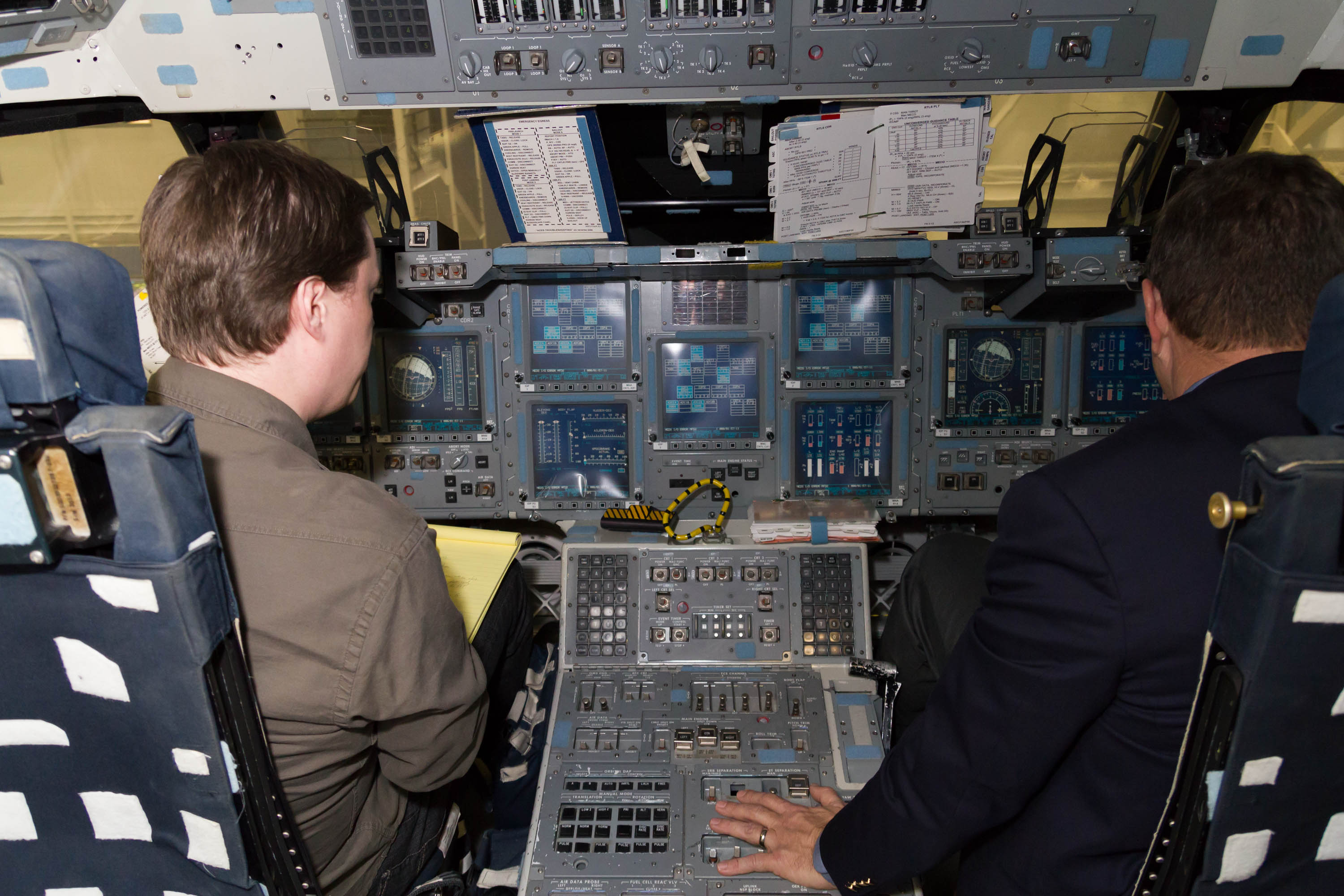The photograph captures the cockpit of a modern jet airplane, likely situated in a hangar given the lack of visible outdoor movement through the windows. Seated in the cockpit are two individuals who appear to be male pilots or trainees in their forties, engaged in performing checks and interfacing with the plane's avionics. The individual on the left, wearing an olive drab dress shirt with black pants, sits in the pilot seat and is taking notes on a yellow notepad. The person on the right, in a dark blue suit with a lighter blue shirt and black dress pants, occupies the co-pilot seat and is actively manipulating instruments with his left hand, which is adorned with a gold ring.

The cockpit is dominated by a variety of instruments, many of which are square screens displaying blue text. The central console, around 20 inches wide, is populated with numerous switches and buttons, highlighting the complexity of the aircraft's controls. Various papers and parts of a manual are taped to the windshield and the upper instrument panel, indicative of a comprehensive checklist procedure being followed. The photograph, devoid of any readable text, exudes an atmosphere of precision and diligence as the pilots ensure all systems meet the necessary requirements.